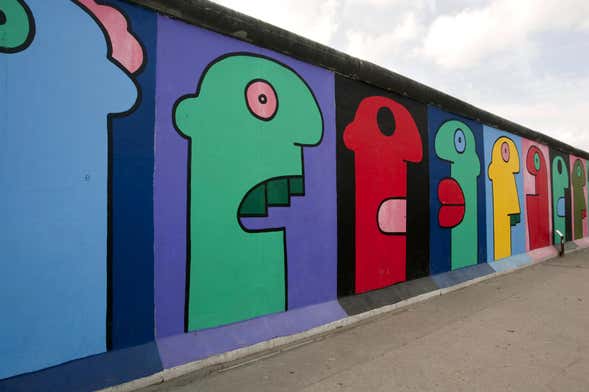The photograph captures a vibrant and playful wall mural painted along a long, plain concrete wall, adjacent to a cement walkway. The mural features multiple cartoon-like profiles of faces in an animated style, each uniquely colored and arranged in a series of colorful squares. Each face profile has a distinctive eye and mouth, with variations in expression; some mouths are open while others are closed. Key details include a face with a purple background and green skin, featuring a yellow eye and visible teeth, another with a red background and black eye, and yet another with a green background, blue eye, and puffy lips. Additional faces include a yellow one with a pink eye and protruding teeth, along with other profiles in various hues of reds and greens. The top of the wall is painted black, and in the upper right corner of the image, a light blue sky with clouds is visible. The colorful array of profiles collectively creates an engaging and cheerful outdoor mural.